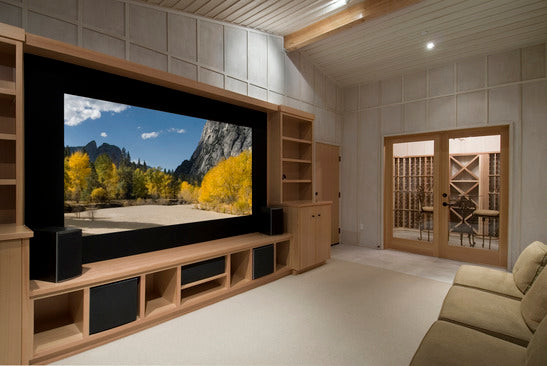This is a detailed indoor image of a sophisticated living room, potentially a 3D render, designed to resemble a small home theater. Dominating the left wall is an enormous widescreen television, nearly 85 inches with a black border, flanked by box speakers on both sides, indicating a high-end 5.1 or 4.1 sound system. Surrounding the TV, except at the very top, are light wooden cabinets. The ceiling is cream-colored, and the top part of the wall transitions into gray acoustic tiles, enhancing the room’s acoustic quality. 

To the lower right-hand corner in front of the TV, there are three cushioned beige or white couches, suggesting a cozy seating arrangement for viewing. On the right wall, there are two wooden framed glass panel doors, possibly leading to an area for storing wine bottles. The room is designed with white walls and a beige rug, giving it a clean, modern feel. This living room appears to be tailored for immersive entertainment experiences, perfect for watching movies or playing video games.